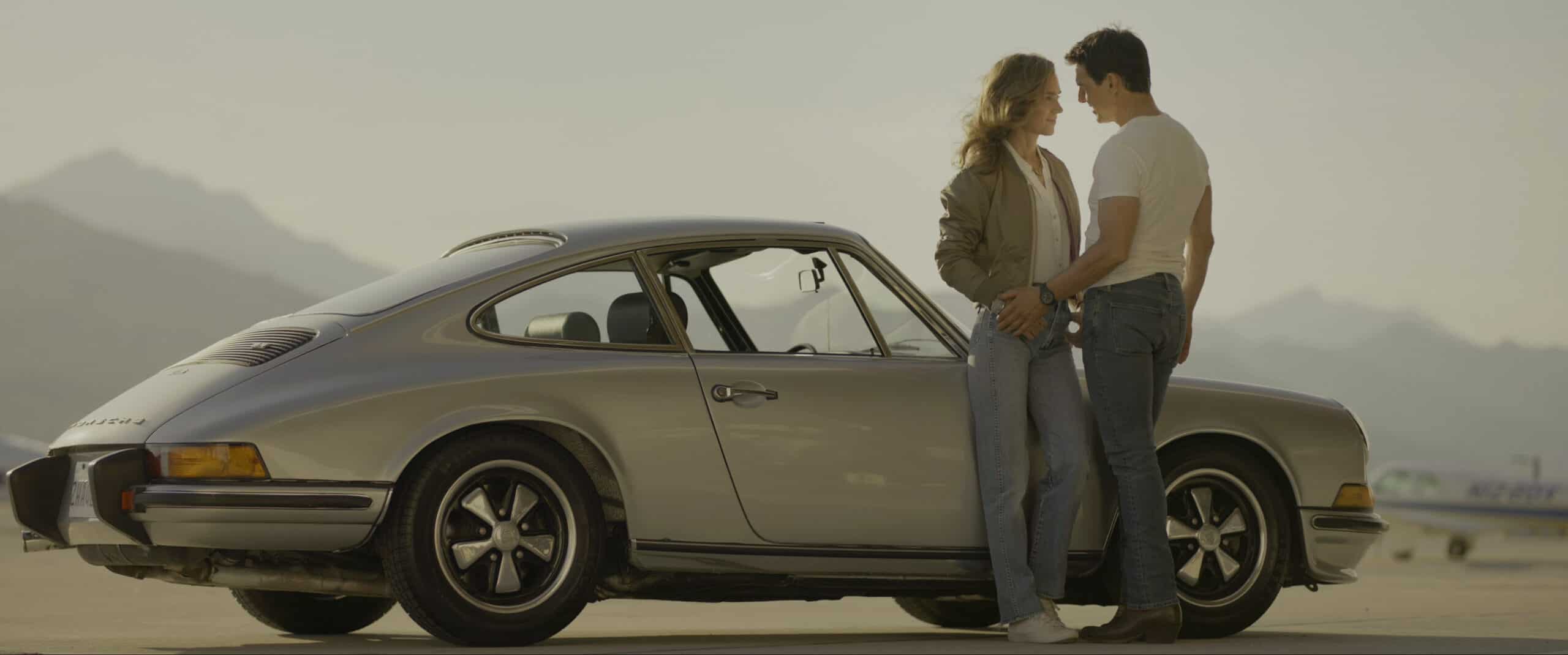The image depicts a couple standing intimately next to a compact silver 1980s-style hatchback car on what appears to be an airline runway. The woman, with long dark blonde hair cascading past her shoulders, is donned in a white shirt, a dull green jacket, light blue jeans, and white sneakers. Standing to her right, the man has short black hair and is dressed in a plain white t-shirt, darker blue jeans, and a black watch on his left arm. They face each other warmly, with the man holding the woman's hand. The car, notable for its rounded trunk and shiny metallic finish, is detailed with black wheels. In the backdrop, albeit slightly out of focus, are faint silhouettes of mountains under a pale blue sky, evoking a desert-like landscape. Additionally, an airplane is visible, adding to the impression that they're on a runway. The atmosphere is somewhat cool and misty, suggesting it isn't particularly hot.